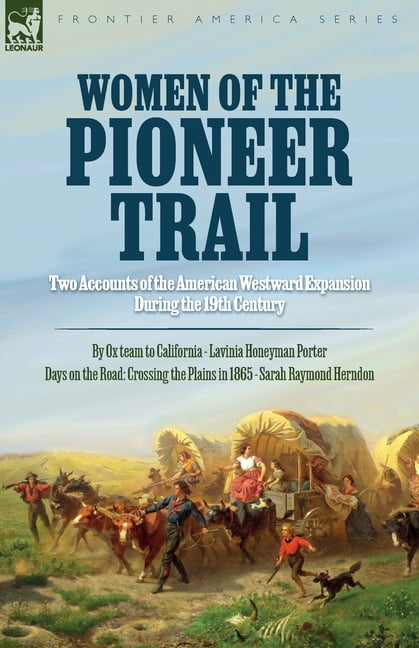This is the cover of a paperback book from the Frontier America Series. The cover showcases a vibrant painting set in the 19th-century American West, highlighting the theme "Women of the Pioneer Trail." At the top right corner, the logo "Lee Onar" is displayed. The title reads, "Women of the Pioneer Trail: Two Accounts of the American Westward Expansion During the 19th Century," followed by the subtitles, "By Ox Team to California, Lavinia Honeyman Porter," and "Days on the Road, Crossing the Plains in 1865, Sarah Raymond Herndon."

The scene depicts three Conestoga wagons traversing a flat, open plains landscape with a faint mound or hill in the background. The central wagon is pulled by oxen and led by a man in a blue shirt and black pants. Inside this wagon, a woman in a red and white dress sits beside a child in a green dress. Another woman inside the wagon hands fabric to a woman walking alongside. Nearby, a child in a red shirt and black pants runs alongside a dog. 

At the bottom right corner, the skeleton of an ox is visible, hinting at the hardships faced during the journey. To the left, another wagon is drawn by mules, led by a man in an orange shirt and brown and gray pants, who is handing a rifle to a woman sitting in the wagon. The sky above them is clear and blue, adding a sense of vastness to the pioneer trail scene.